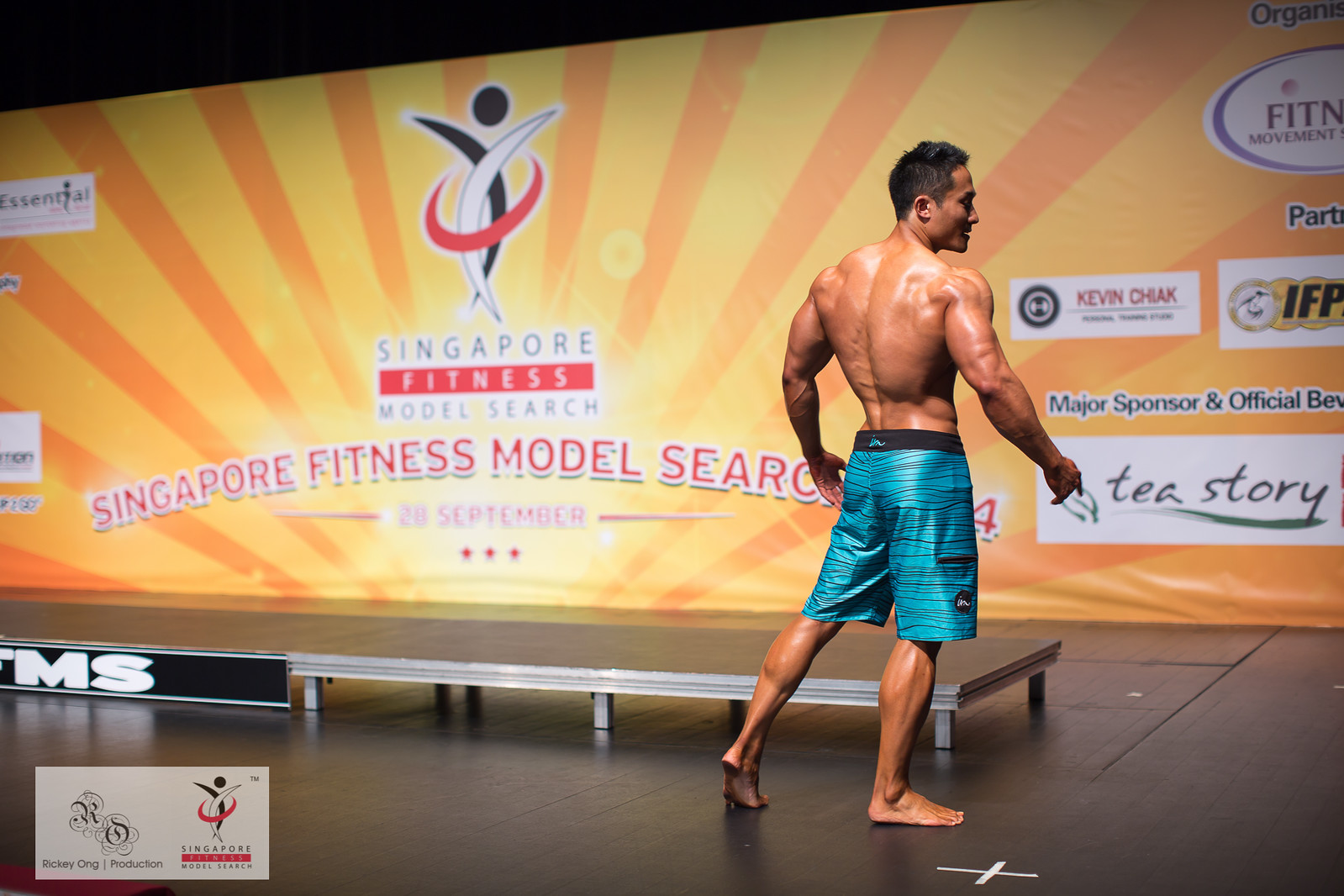The image captures a highly detailed scene of a muscular man participating in the Singapore Fitness Model Search contest. Positioned with his back to the camera, the man, shirtless and wearing turquoise blue shorts with a black waistband, appears to be posing slightly to the side. His well-defined calves and strong build are prominently displayed. He stands barefoot on a brown tiled floor, possibly in a gym or conference center, with a short stage in front of him.

The background is dominated by an expansive poster, stretching from one end to the other, featuring bold, vivid colors—predominantly oranges and yellows. At its center, the poster prominently displays the words "Singapore Fitness Model Search" in red letters accented with white and blue highlights. The emblem, located in the middle, depicts a black and white crescent moon and a sun with rays extending from it.

Additional details include advertisements for event sponsors scattered across the poster. For instance, "T-Story" appears on the left side in large letters, accompanied by various logos and text indicating sponsorships, though some parts are obscured by the contestant. The flooring has markings, including a taped "X."

The man stands on a smaller stage section that is black with silver accents and displays a white "X." Other visible elements on the poster include September 20th in red, three red stars, and various other symbols and text in black, red, and white, highlighting additional sponsors like "IFP" and names like "Kevin Schick."

Overall, the image is a dynamic snapshot of the fitness modeling contest, showcasing both the contestant's physique and the vibrant promotional materials surrounding the event.